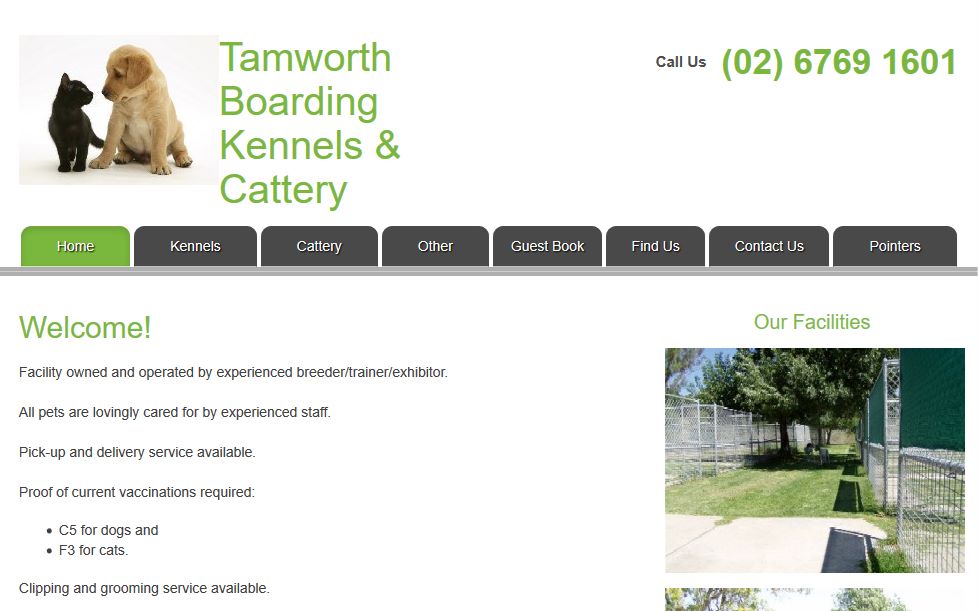The front page of a kennel and cattery boarding website is displayed. At the top right, a heartwarming image features a yellow Labrador puppy gazing at a black kitten. To the left of this image, the business name "Tamworth Boarding Kennels and Cattery" is prominently written in a light lime-green font. 

Further left, in small black font against a white background, is the phrase “Call Us” followed by the phone number (02) 679-69-1601 in the same lime-green color. Beneath this line are the website navigation options. The "Home" option, highlighted in green, is at the far right. Moving leftwards, the remaining options "Kennels," "Cattery," "Other," "Guest Book," "Find Us," "Contact Us," and "Pointers" are displayed with white text on a black background.

Below the navigation menu, in green text, is the welcoming message "Welcome," followed by "Family Owned and Operated Experience Breeder Trainer Exhibitor" in black font. The next line reads, "All pets are lovingly cared for by experienced staff." Below this, more information is provided in black text: "Pickup and Delivery Service Available, Proof of Current Vaccinations Required," with two bullet points listing "C5 for Dogs" and "F3 for Cats." Further services such as "Clipping and Grooming Services are available" are highlighted.

To the left of this information, under the "Contact Us" and "Pointers" tabs, there is a picture of the facility. The image showcases a grass field, some concrete paving, a surrounding fence, and a couple of trees in the background, providing a glimpse into the pleasant environment where the pets are cared for.